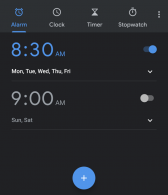The image depicts a user interface for a clock application with a predominantly blue and gray color scheme. At the top, there is a gray rectangle with the word "Alarm" prominently displayed, indicating the current function of the app. Below, there are several icons representing different functionalities: a clock, a timer, and a stopwatch. 

A visible column showcases a digital readout highlighting "8:30 AM" in blue, with the days "Monday, Tuesday, Wednesday, Thursday, Friday" listed underneath, also in blue. There is a drop-down menu that reveals "9 AM" alongside the days "Sunday" and "Saturday." Another drop-down menu demonstrates the application's options but remains untoggled. 

The background is uniformly gray, providing a neutral backdrop to the colorful elements. At the bottom of the interface, a blue circle with a white cross at its center serves as an additional interactive button. The text throughout the image is blurry with pixelated edges, rendering words like "alarm," "clock," "timer," "stopwatch," "8:30 AM," and the days of the week just discernible.